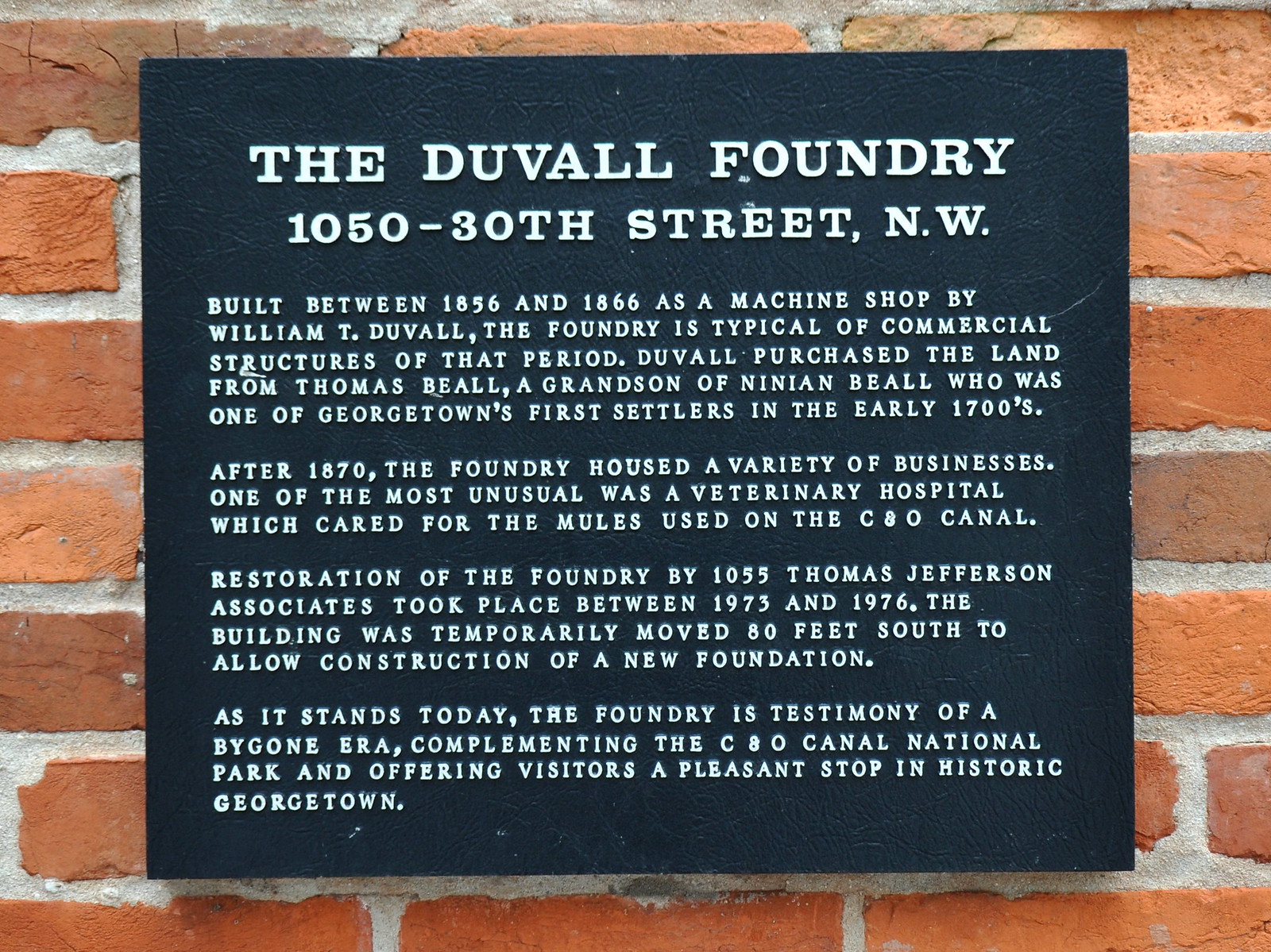The image depicts a black commemorative plaque with white text, affixed to a brick wall composed of reddish-brown bricks interspaced with cement. The plaque reads:

"The Duval Foundry
1050 30th Street, NW

Built between 1856 and 1866 as a machine shop by William T. Duval, the foundry is typical of commercial structures of that period. Duval purchased the land from Thomas Beall, a great-grandson of Ninian Beall, one of Georgetown's first settlers in the early 1700s. After 1870, the foundry housed a variety of businesses, including a veterinary hospital that cared for the mules used on the C&O Canal. Restoration of the foundry by 1055 Thomas Jefferson Associates took place between 1973 and 1976. The building was temporarily moved 80 feet south to allow for the construction of a new foundation. As it stands today, the foundry is a testimony to a bygone era, complementing the C&O Canal National Park and offering visitors a pleasant stop in historic Georgetown."

The plaque is a testament to the historical significance of the Duval Foundry, highlighting its origins, diverse uses over time, and eventual restoration. The background of the scene features the richly textured brick wall, providing a vivid backdrop to this piece of Georgetown's heritage.